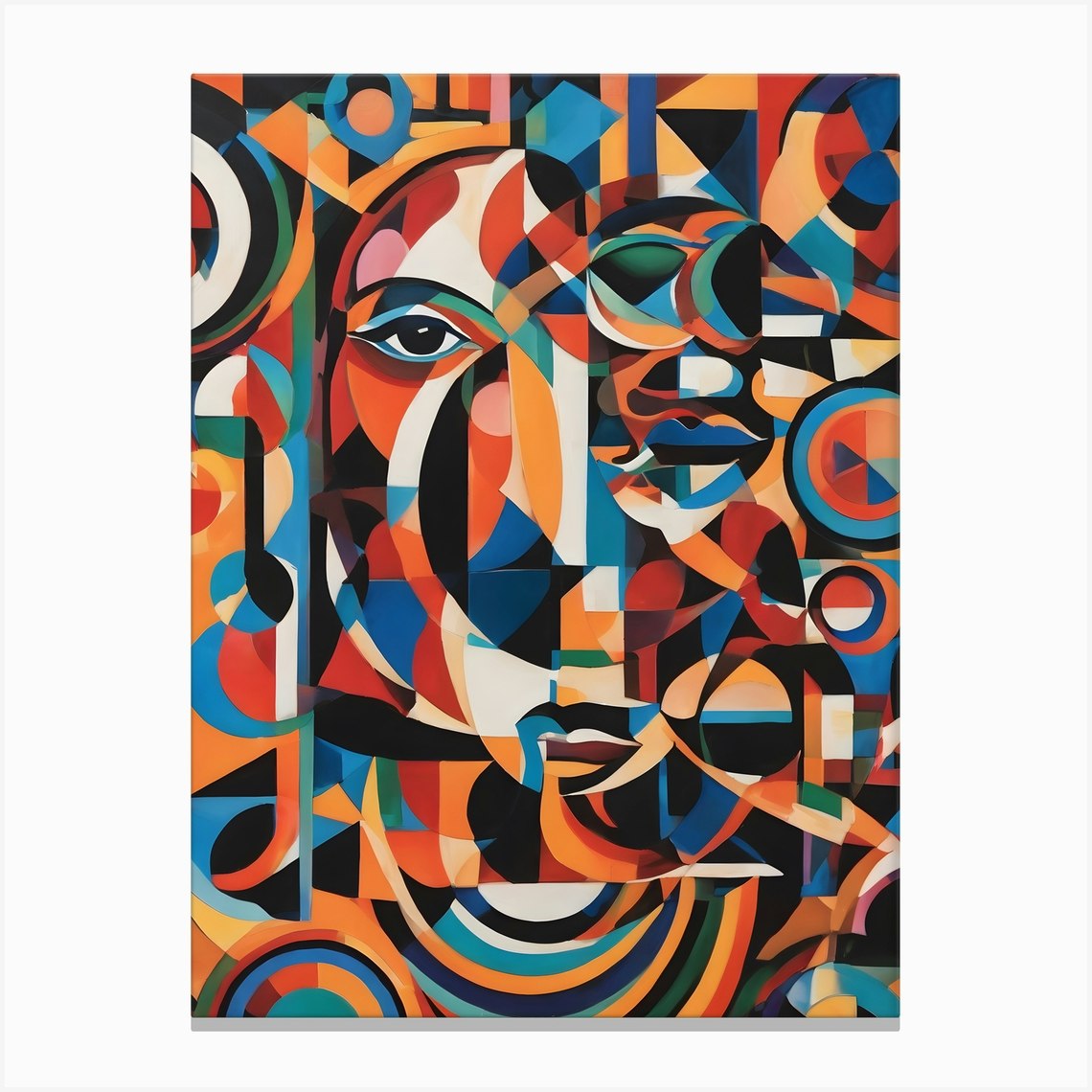This abstract painting, displayed on a white wall, features a vivid composition of geometric shapes and vibrant colors, including muted yet rich tones of yellow, red, brown, black, white, blue, and green. The artwork is centrally positioned within an off-white border that frames it—comprising approximately 15-20% on the sides and 5-10% on the top and bottom—giving it a portrait orientation that is significantly taller than it is wide. Dominating the piece is the fragmented depiction of a woman's face, where an eye is discernible in the upper left and lips in the lower right. The face, along with the shoulders, is segmented by various overlapping shapes, including swirls, curves, edges, and triangles, creating a mosaic of multicolored sections. The right side of the face appears more densely packed with shapes and detail, enhancing the intricacy of the composition. The entire artwork is bathed in a spectrum of colors reminiscent of a full Crayola crayon box, yet the hues remain striking without being overly bright or garish. Shadows cast by the canvas onto the wall hint at the depth and textural reality of the piece.